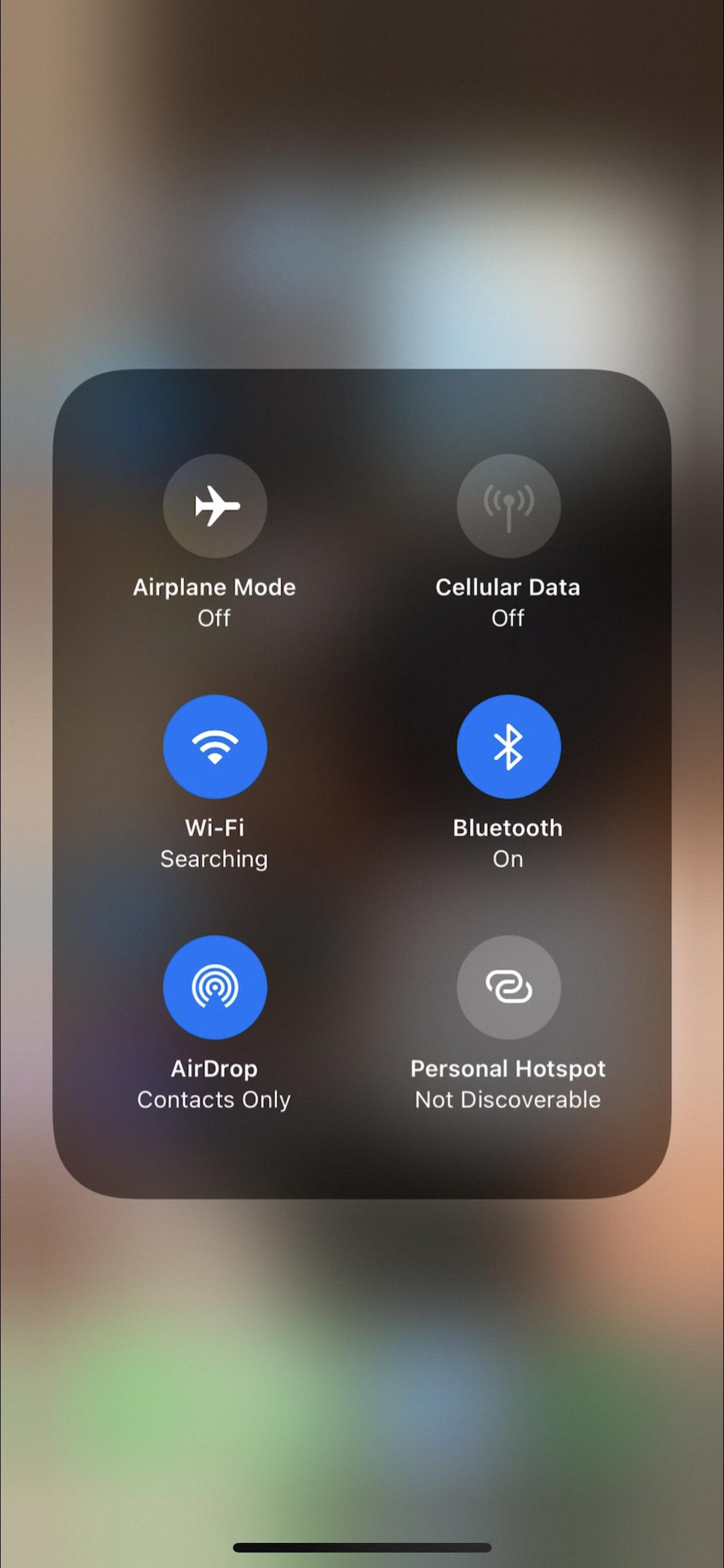This image displays a cell phone screenshot in portrait orientation, with a length at least twice its width. The backdrop is intentionally blurred to direct attention to a central pop-up window. This pop-up, a vertical rectangle with rounded corners, houses two columns of icons, each containing three items.

Starting from the top left, the first icon is a gray circle featuring a white airplane symbol, labeled "Airplane Mode Off." Below it is a blue circle with a white Wi-Fi signal icon, labeled "Wi-Fi Searching," followed by another blue circle featuring blue semi-circles, labeled "AirDrop Contacts Only."

On the right-hand side, the top icon displays a cell signal graphic within a grayed-out bubble, labeled "Cell Data Off." Directly underneath, a blue bubble with a white Bluetooth icon indicates "Bluetooth On." The final icon in this column is a gray bubble with a chain link graphic, labeled "Personal Hotspot Not Discoverable," which is also grayed out.

It appears that the intention behind this screenshot was to capture the various connectivity settings on the phone.